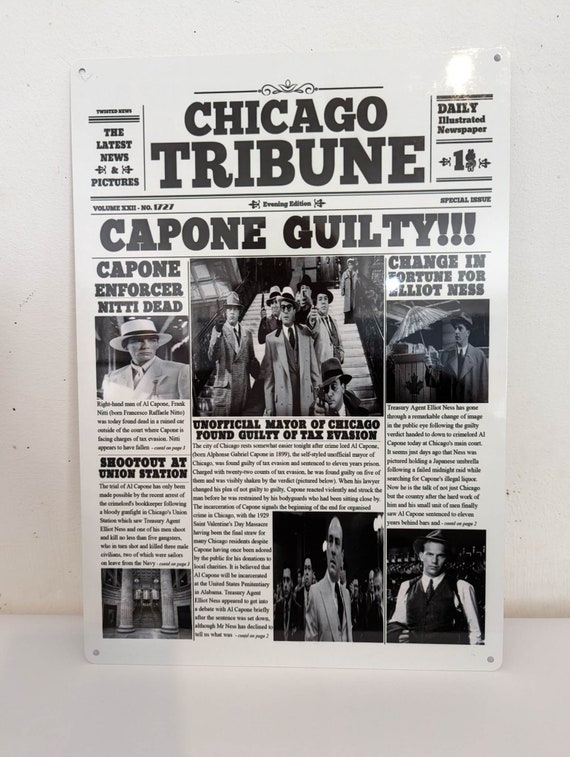This is an old cutout of a front page from the Chicago Tribune newspaper, sitting on a white background and a white table. The newspaper, dated to the time of Al Capone's conviction, features multiple stories related to the infamous mobster era. The bold headline proclaims "Capone Guilty," with the sub-headline "Unofficial Mayor of Chicago Found Guilty in Tax Evasion" beneath it. To the left, a story is titled "Capone Enforcer Nitty Dead" and another submission, "Shootout at Union Station." On the right side, there is a piece titled "Change in Fortune for Elliot Ness." Titled prominently at the top, the newspaper is indicated as a "Daily Newspaper One Cent" with "The Latest News and Pictures" on the top left corner. This laminated cutout has been mounted on a board with clear tacks and has a slightly glossy appearance, despite typical newspapers being matte. It offers a snapshot of a turbulent time in Chicago's history, presented in black and white.